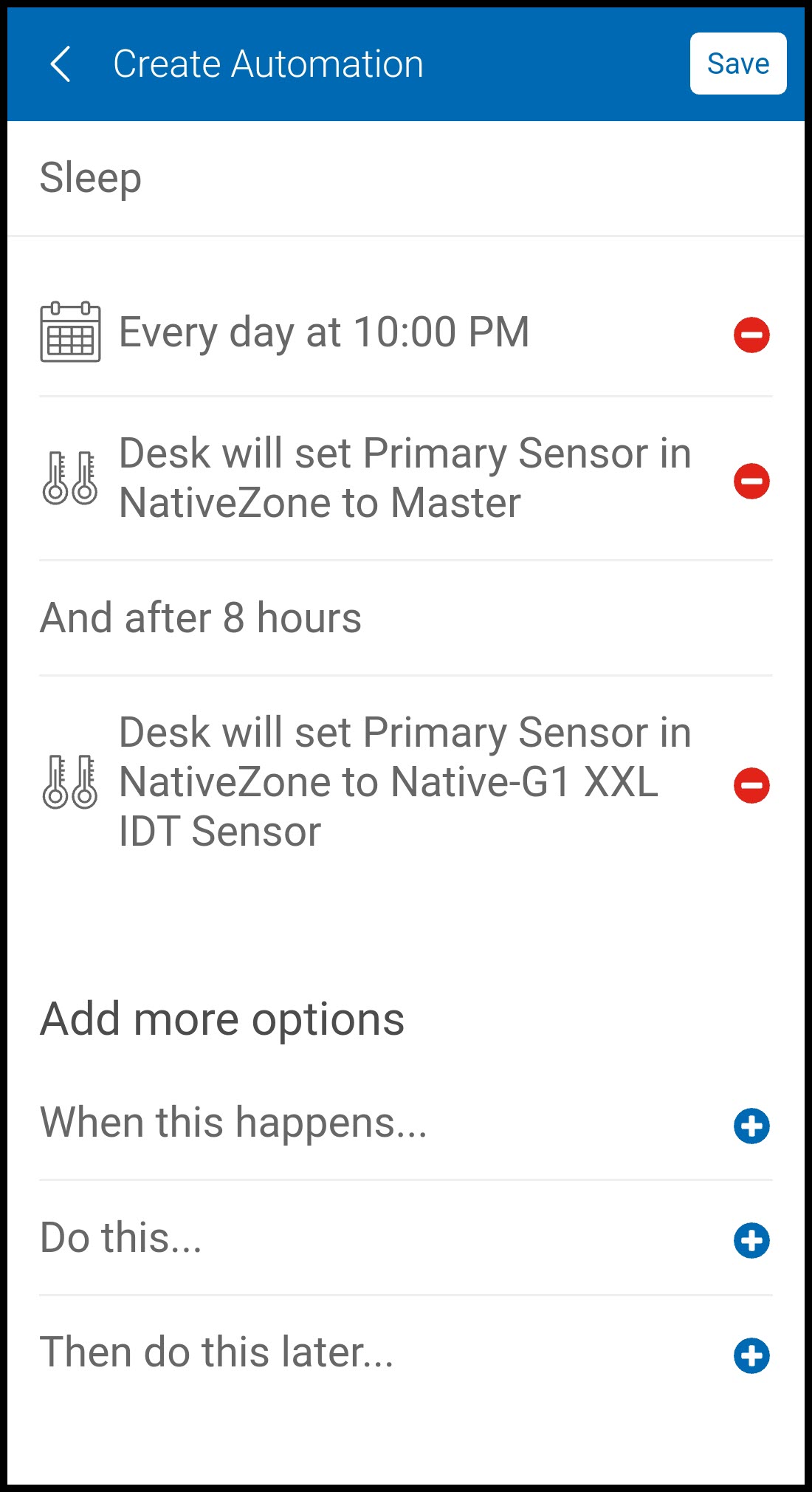**Detailed Caption:**

In this screenshot, a blue bar stretches across the top of the screen. On the left side of this bar, there's a small arrow pointing to the left. Next to the arrow, the text "Create Automation" is written in white. On the right side of the top bar, there's a small white "Save" button.

The rest of the screen has a white background. Along the left margin, the word "Sleep" is displayed. Below it, there's an image of a calendar, accompanied by the text "Every day at 10 p.m." next to a red circle with a minus sign in it. Further down, there is a statement that reads "Desk will set primary sensor in native zone to Master," also with a red circle containing a minus sign. 

Underneath that, the text continues with "And after eight hours," followed by another line, "Desk will set primary sensor in native zone to native G1 XXL IDT sensors," accompanied by a red circle with a minus sign. 

At the very bottom of the screen, there's an option to "Add More Options." Under this header, there are three separate sections:
1. "When this happens," marked with a blue circle containing a plus sign.
2. "Do this," also signified by a blue circle with a plus sign.
3. "Then do this later," with the same blue circle and plus sign.

Each of these three sections has an ellipsis (three dots) at the end of the text, indicating further options or settings.